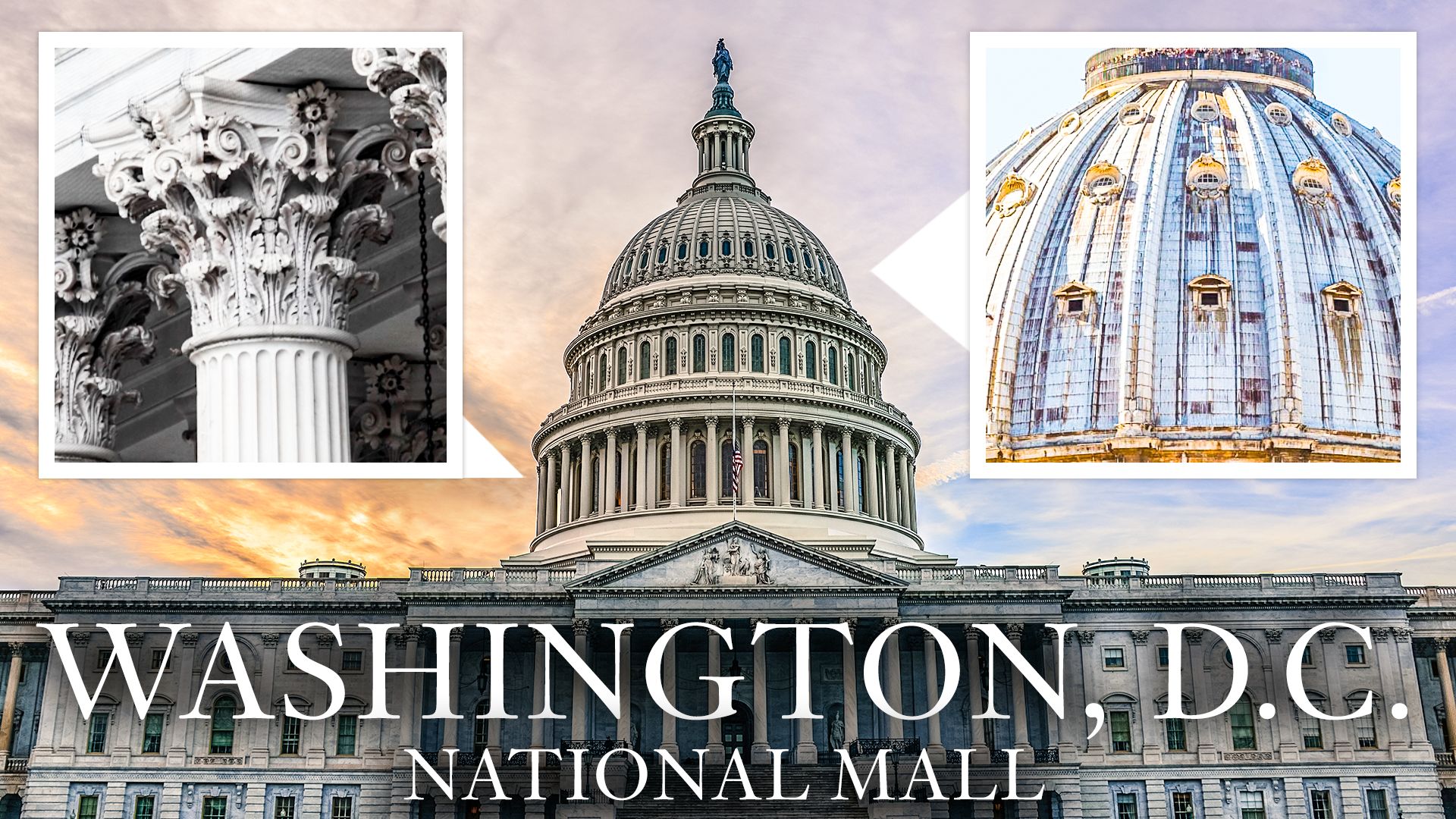A visually captivating graphic prominently features the iconic white dome and pillars of the Capitol Building with the text "Washington, D.C. National Mall" in bold white lettering at the bottom. The main image showcases the Capitol under a striking sky decorated with blue and adorned with hues of orange and yellow, possibly capturing the sun's glow. Flanking the central image are two smaller, detailed insets. On the left, a close-up photograph reveals the intricate designs and craftsmanship of the Capitol's ornate pillars. On the right, a closer view of the Capitol Dome highlights the individual panels and windows, complete with natural patina and weathering, offering a glimpse into the architectural grandeur and historical depth of this monumental structure.